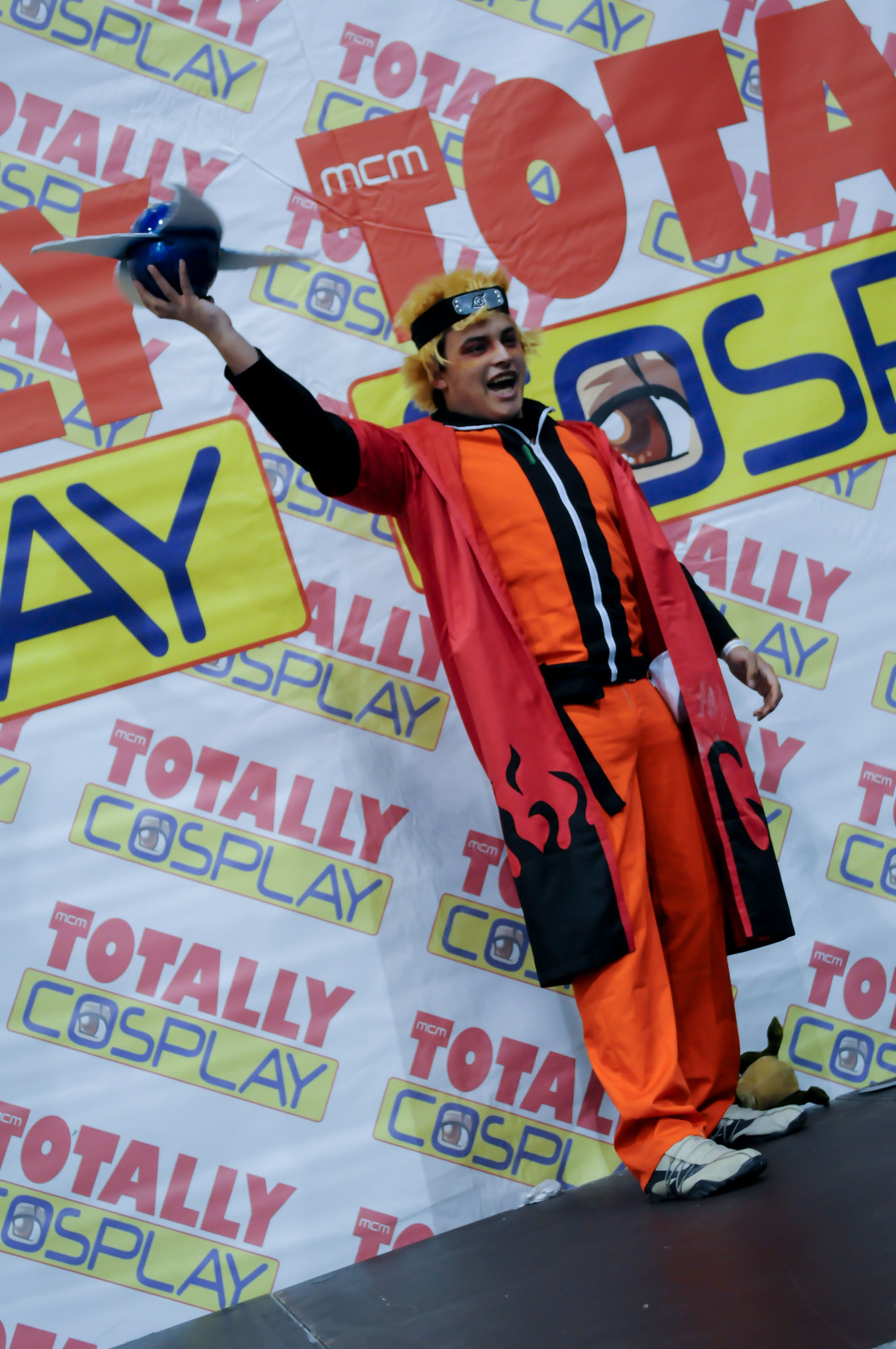The digital photograph captures a man in an elaborate costume standing indoors in front of a large poster or tarp repeatedly displaying the words "Totally Cosplay" in various diagonal orientations. Centered in the image, the man features platinum blonde hair and a small mustache, with a distinctive black headband adorned with a white design. His costume comprises orange pants, an orange zippered jumpsuit, a striking red overcoat decorated with black flames at the bottom, and a black long-sleeved shirt peeking out from beneath his overgarments. He cheers open-mouthed, holding a mysterious flying device or creature with grey wings and a grey tail high above his head, while his other hand remains by his side. Completing his look, he wears white sneakers.